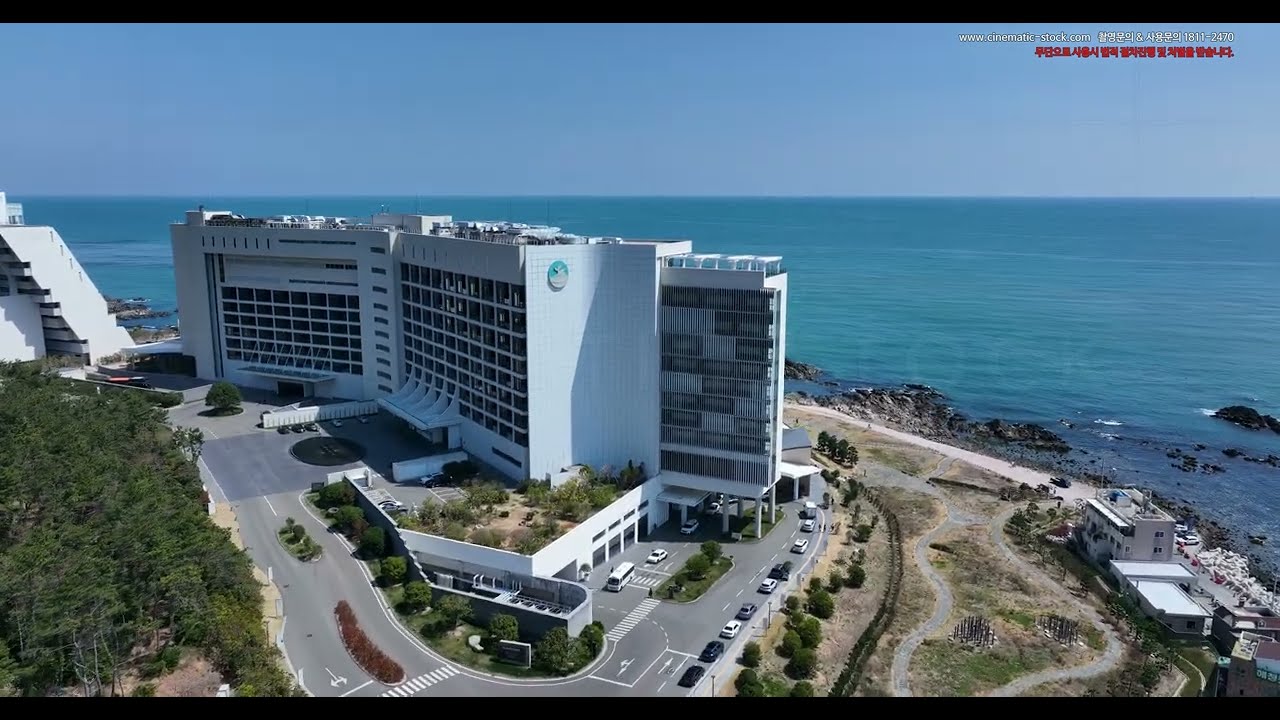This aerial photograph captures a striking white hotel situated on a pavement and surrounded by greenery and shrubs in the foreground. The hotel, featuring three distinct wings or sections, presents a tiled exterior with square, almost rectangular windows and rises approximately eight stories high. Clearly designed with aesthetic appeal, it includes a rooftop bar and multiple entrances, with cars and buses visible around the premises.

To the left of the hotel, there is a smaller white-brick building, possibly a house, set amid green areas with rocks and shrubs. The hotel is strategically positioned on the edge of rocky cliffs, overlooking an expanse of turquoise ocean water. The ocean stretches out behind the rocky shoreline, meeting the clear blue sky on the horizon.

The image also includes commercial elements, with the upper right bearing watermarks: "www.cinematic-stock.com" along with white and red Korean text, and "1811-2470". The logo of the building is a turquoise circle pattern, heightening its distinctive character. The photo, likely taken on a clear, sunny day, captures the serene ambiance of this beachside locale perfectly, despite the absence of a sandy beach.